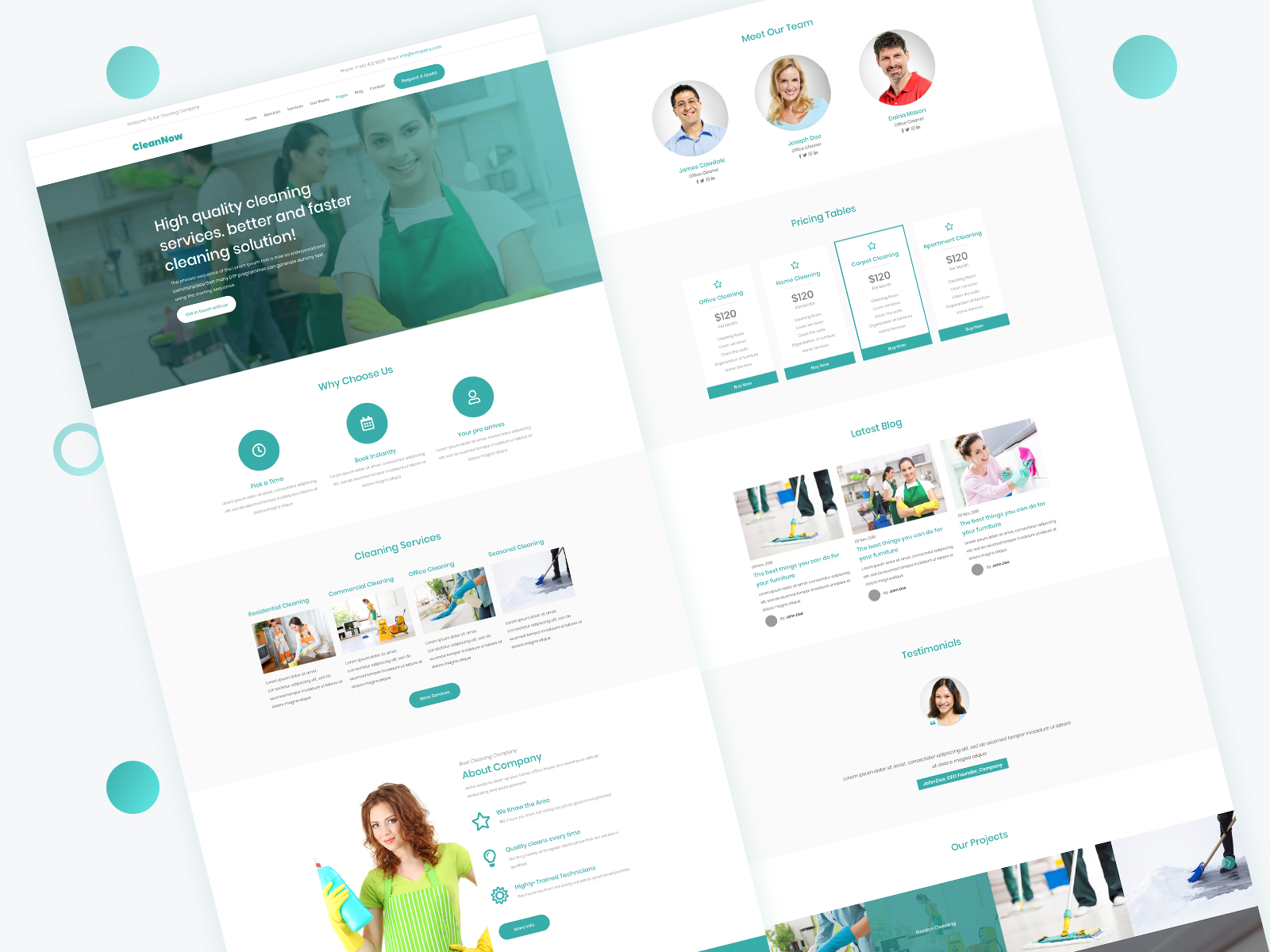The screenshot captures an image of a professional house cleaning service website. The top of the page prominently displays the slogans "High Quality Cleaning Services" and "Better and Faster Cleaning Solutions." The website features a visual layout with various images, including individuals dressed in aprons suggesting professionalism and readiness to work. In one image, a smiling young woman stands out, though the picture is too small to see her clearly. The website appears to offer multiple service plans, which seem to be priced around $20, $50, and $100, though the exact amounts are difficult to discern due to the small text. Additionally, the site includes images of people performing cleaning tasks, including one person holding a cleaning rag or sponge, and another mopping the floor in an image located near the bottom of the page. The overall impression is that the website allows customers to hire cleaning services efficiently and conveniently.